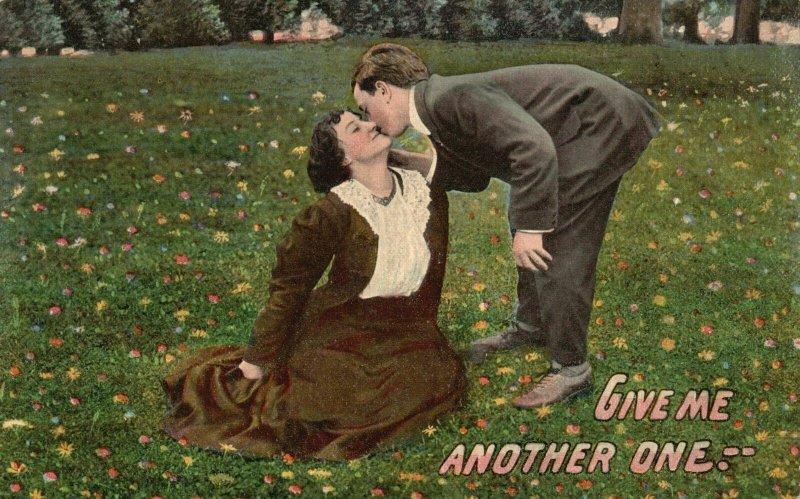In this vintage-style artwork, a mother and her young son share a tender moment in a vibrant field of colorful flowers. The mother, wearing a long brown dress with a white lace bodice, sits gracefully on the lush grass, her legs concealed beneath her attire. Her brown hair cascades gently as she looks up adoringly at her son. The little boy, dressed in a black suit with a white shirt and brown shoes, bends down to plant a loving kiss on her cheek. The serene background is adorned with trees, offering a tranquil setting to the affectionate scene. In the bottom right corner of the image, handwritten text whimsically reads, "Give Me Another One," set in pink letters outlined in black. The overall piece exudes a nostalgic charm, enhanced by delicate floral accents dotting the verdant grass and a subtle hint of vintage photographic touch-up.